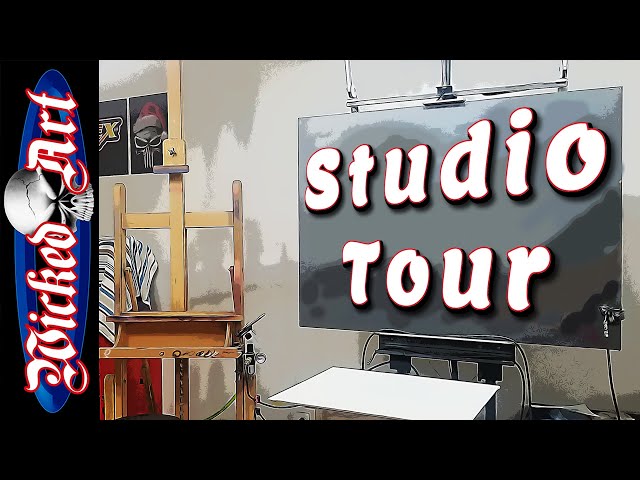This highly detailed indoor scene has the stylistic precision of a photographic image. The setting prominently features a silver metal stand holding a gray canvas or print, with the words "Studio Tour" painted in white text on it. In front of this stand is a small white table, approximately the size of a desk, with a couple of wires hanging down. To the left of the main canvas, there's an old-fashioned brown wooden easel, noticeably lacking a painting.

Adding to the atmosphere, the top left corner of the image showcases a poster featuring a skull-themed Santa Claus beneath the letter "X". Adjacent to this on a chair is a blue and white-beige towel draped over. The left-hand side of the image is visually dominated by the text "Wicked Art" in a fancy white font with a red border, vertically oriented along the side. This text is accented by a graphic skull positioned between the words "Wicked" and "Art", all set against a blue oval.

Completing the scene are rectangular black bars across the top, bottom, and left edges of the image, giving it a screenshot-like appearance, possibly from a YouTube video. The background is a grayish wall, adding a subtle backdrop to the overall composition.